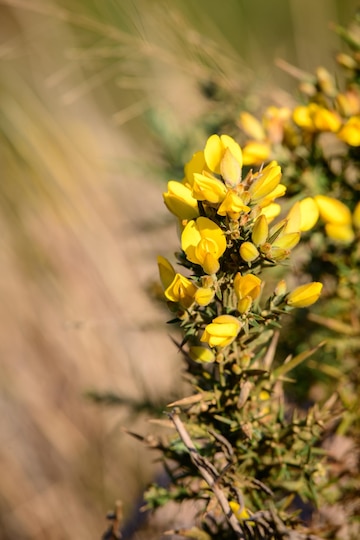The image captures a cluster of bright yellow flowers with small, somewhat closed buds, prominently displayed on the right-hand side. These flowers have green and occasionally brown stems that appear slightly spiky and jumbled. The background is a complete blur, showcasing hues of green and brown, giving off an impression of motion or a sun-drenched, dry environment—almost like an army olive green color. The scene appears natural and unkempt, suggesting these flowers might be growing wild, possibly along the side of a road, rather than in a tended garden. Tall, out-of-focus grass and additional yellow stalks reminiscent of reed branches enhance the rustic feel of the setting. The overall focus remains on the vibrant, sunlit flowers, with any background details purposefully blurred to draw attention to the striking yellow cluster in the foreground.